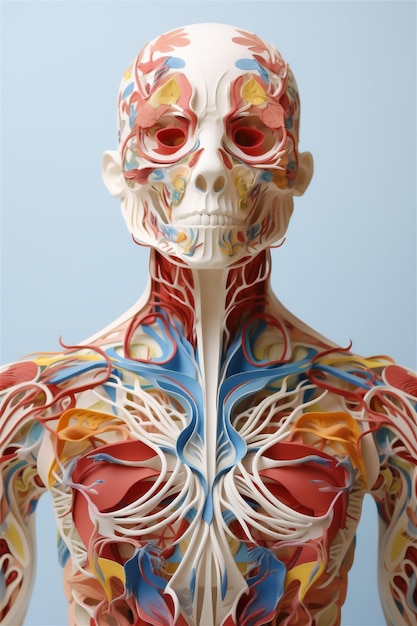The image depicts an intricate, multicolored anatomical model of the human upper body, likely for educational purposes or artistic representation. Centered against a light blue background, the model showcases an artistic blend of skeletal and anatomical elements. The skull is adorned with red tissue around it, featuring two rows of red paper-like structures for the eyes and flower-like blue and white petals attached on top. The nose displays minimal detail, having two red spots on either side of the bridge. The mouth area highlights vibrant white, blue, and orange spots near the upper and lower jaws, with a predominantly red neck suggesting muscles. 

The chest area is designed with blue elements representing veins, fanning out intricately and turning white, almost resembling filigree. While the heart isn't visible, the chest features two large structures that could represent lungs, surrounded by decorative strings and frills. Yellow and green hues are present, symbolizing nerves and ligaments respectively. The overall presentation suggests an interplay between a detailed anatomical reference and an artistic creation, combining educational detail with a visually captivating, almost paper-crafted aesthetic.